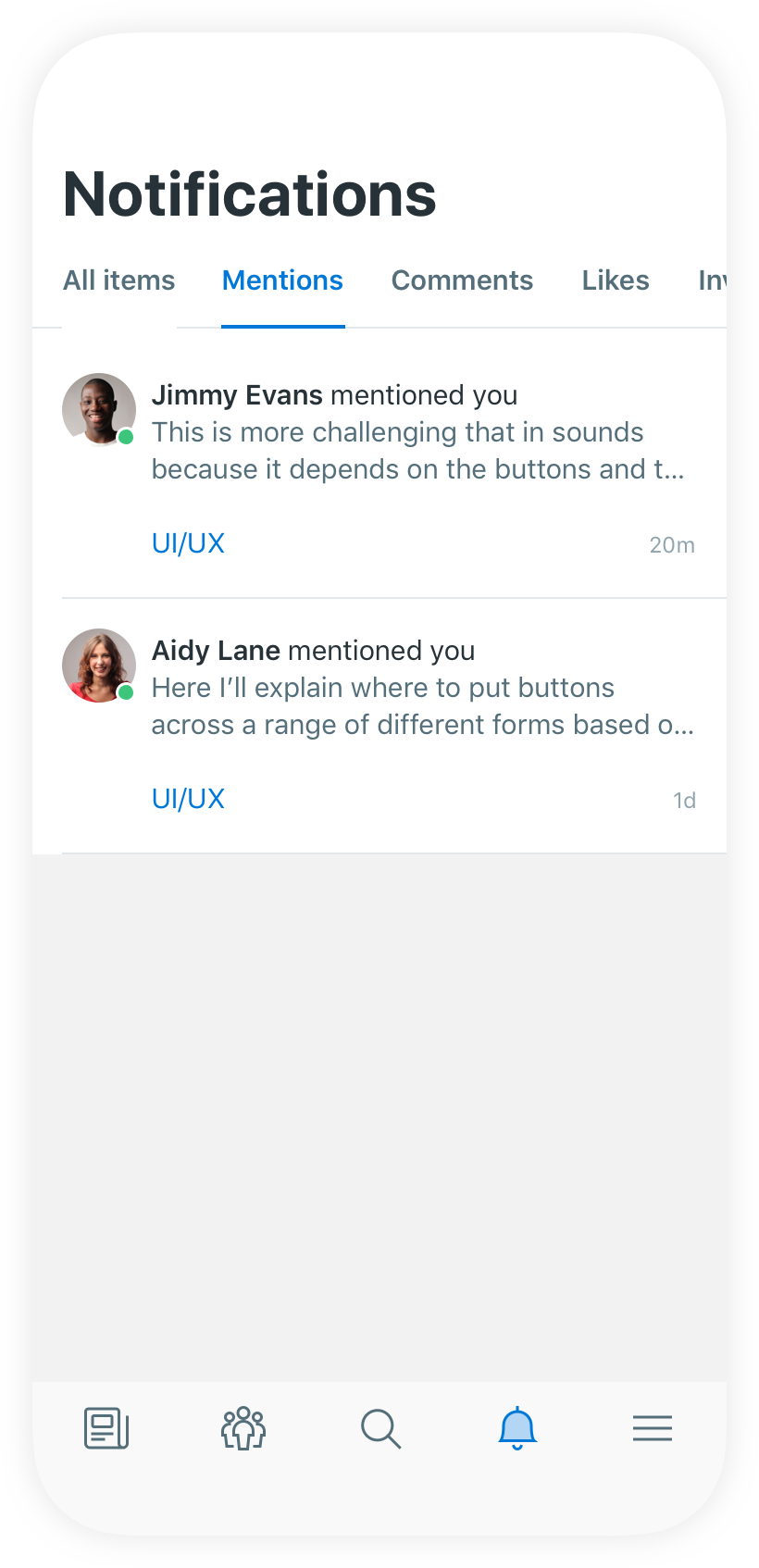In this image, the notification screen is prominently displayed. The title "Notifications" is written at the top in black text against a white background. Below the title, there are several tabs: "All Items," "Mentions," "Comments," "Likes," and "Invites." These tabs are written in dark gray, except for "Mentions," which appears in blue and is underlined, indicating it is the currently selected tab.

The first notification is from Jimmy Evans, stating, "Jimmy Evans mentioned you: This is more challenging than it sounds because it depends on the buttons and the text." The text "UI/UX" is written in blue, suggesting a clickable link or category. Jimmy Evans' profile shows a green dot, indicating he is online, and the notification was received 20 minutes ago.

The second notification is from Adelaine, reading, "Adelaine mentioned you: Here I'll explain where to put buttons across a range of different forms." Similarly, the text "UI/UX" is highlighted in blue. Adelaine's profile is also marked with a green online status dot, and this notification was received one day ago.

At the bottom of the screen, there are navigation buttons for "Notifications," "Search," "Groups," "Feed," and "Settings." These buttons are in gray, except for the "Notifications" button, which is in blue, indicating it is currently active.